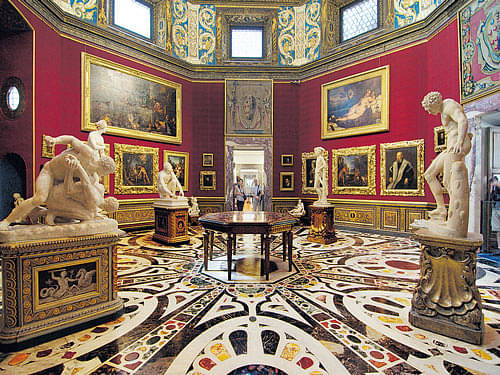The room, likely a gallery in a museum, exudes opulence and sophistication. Hexagonal or possibly octagonal in shape, it features red walls adorned with an array of large portraits and paintings, each encased in grand gold frames. The walls are further embellished with blue and gold ornate details between the windows on the upper section. A gold-painted baseboard runs waist-high along the perimeter, complementing the richly colored walls. In the corners of the room stand four life-size, marble-like sculptures that appear to depict naked figures, reminiscent of classical Greek style. These sculptures are elevated on podiums. At the very center of the space, there's a small octagonal-shaped table. The floor is a striking mosaic of geometric patterns in white, black, yellow, and red, featuring radiating black lines and circular designs. Adding to the scene, a few visitors are seen walking around, taking in the blend of sculptures and paintings that decorate this lavish room.